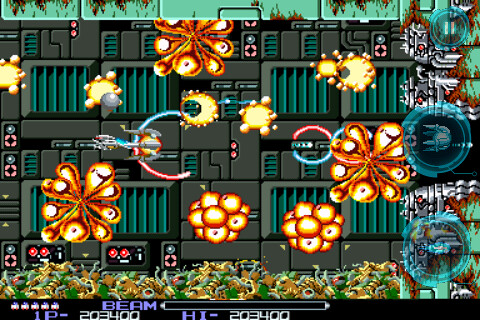The image appears to be a screenshot from a classic space-themed video game. The central focus is on a spaceship, likely controlled by the player, situated on the left-hand side of the screen. This spaceship, presumably the protagonist or "good guy" ship, is actively engaged in combat, firing projectiles towards enemies. Surrounding the main ship are several orange explosions or similar effects, indicating ongoing battles or attacks that the player must dodge. The background is a moody blend of gray and green, depicting the vastness of space.

On the right-hand side of the image, there are bluish bubbles with objects inside them, suggesting either power-ups or obstacles the player must interact with. Additionally, various grayish machines with distinct red spots are visible, potentially serving as enemy crafts or structures within the game.

At the bottom of the image, the user interface displays crucial game information. The text "1P 203400" indicates the player's score, while "BEAM" in purple likely represents the type of weapon currently in use. The high score, also "203400," is displayed, suggesting this might be the player's best performance so far. This information is presented against a dark, almost black UI background, ensuring it stands out clearly for the player.